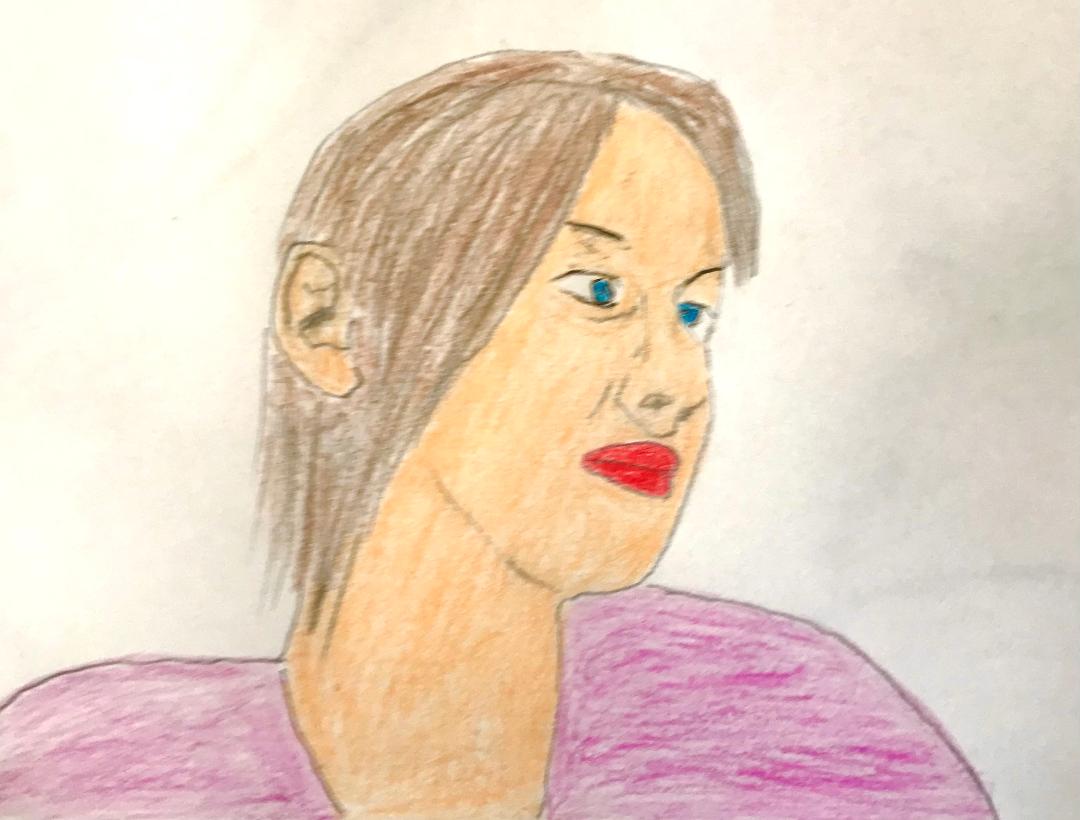This drawing, rendered on a piece of sketch paper, vividly portrays the upper portion of a woman. The illustration focuses from her shoulders and part of her neck upward. The woman's body faces towards the viewer while her head is turned to the right, providing a clear view of the right side of her face and a partial glimpse of the left side. She is depicted wearing a purple top, with the fabric subtly visible. The artist utilized colored pencils, adding depth and dimension to her appearance. Her striking blue eyes bring an element of life to the sketch. She has brown, almost shoulder-length hair, through which her right ear is partially visible.